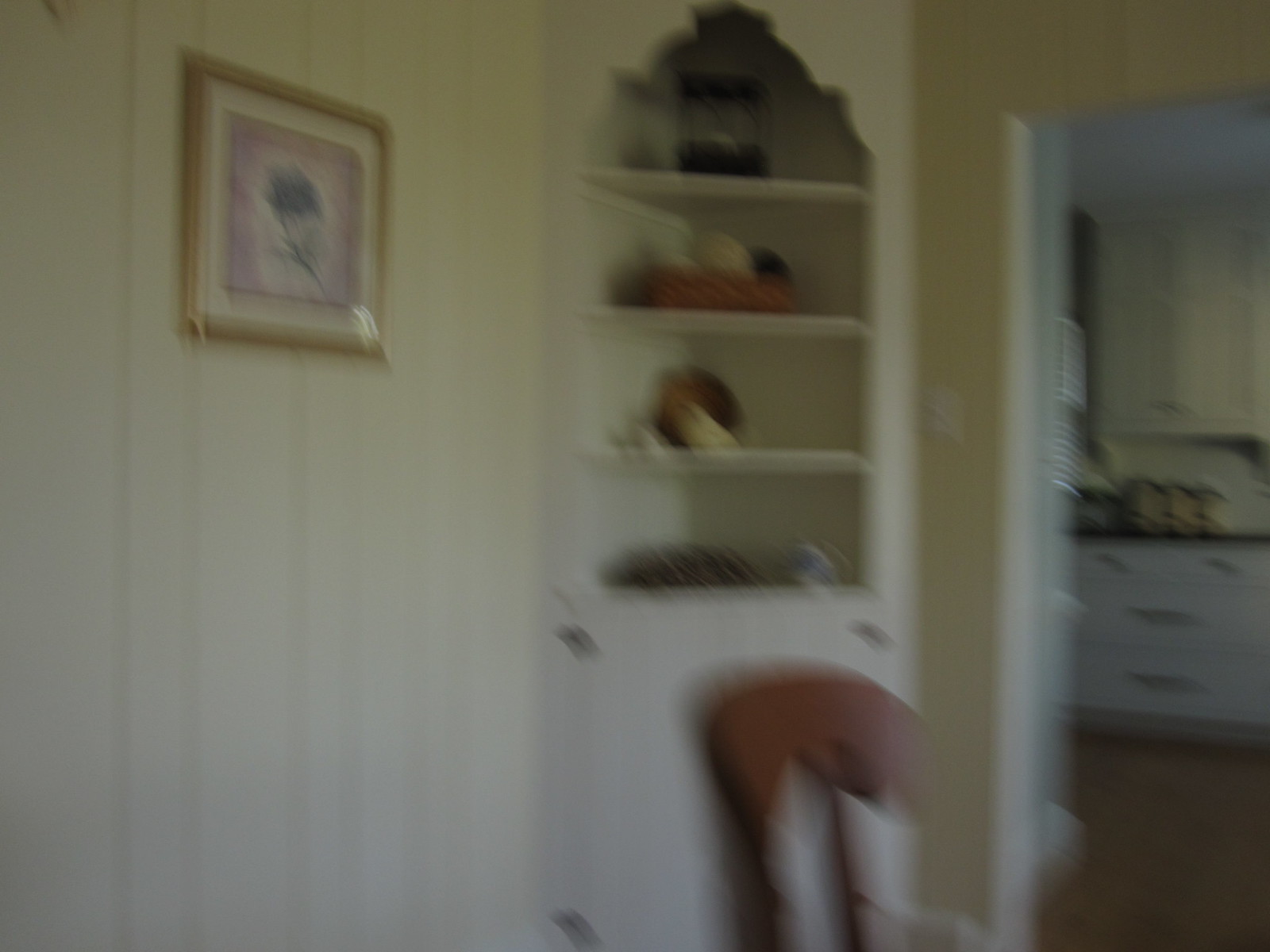This photograph, though very blurry, captures a cozy farmhouse-style interior, characterized by its cream-colored, vertical wood-paneled walls. Central to the image is a charming corner shelf unit, painted a bright white, which stands out against the creamy background. The shelves feature three to four levels and are adorned with various indistinct items, including a wicker basket that seems to hold round objects—possibly spools of yarn. Below the shelves, a hinged door likely opens laterally for additional storage.

In the foreground, we glimpse a high-back wooden chair, probable to be a kitchen chair, with vertical support slats, although the blurriness obscures fine details. Positioned to the right of the corner shelf, there’s a small rectangular cutout on the wall, likely a power outlet.

Beyond the immediate focus of the corner shelf and chair, through a wide archway, is a peek into the kitchen. This adjacent area showcases white cabinets and drawers, a black countertop lined with assorted containers, and a section of pale stained wooden flooring, all contributing to the warm, rustic feel of the home. On the left side of the photo, partially visible, hangs a piece of artwork further enhancing the room’s decorative elements.